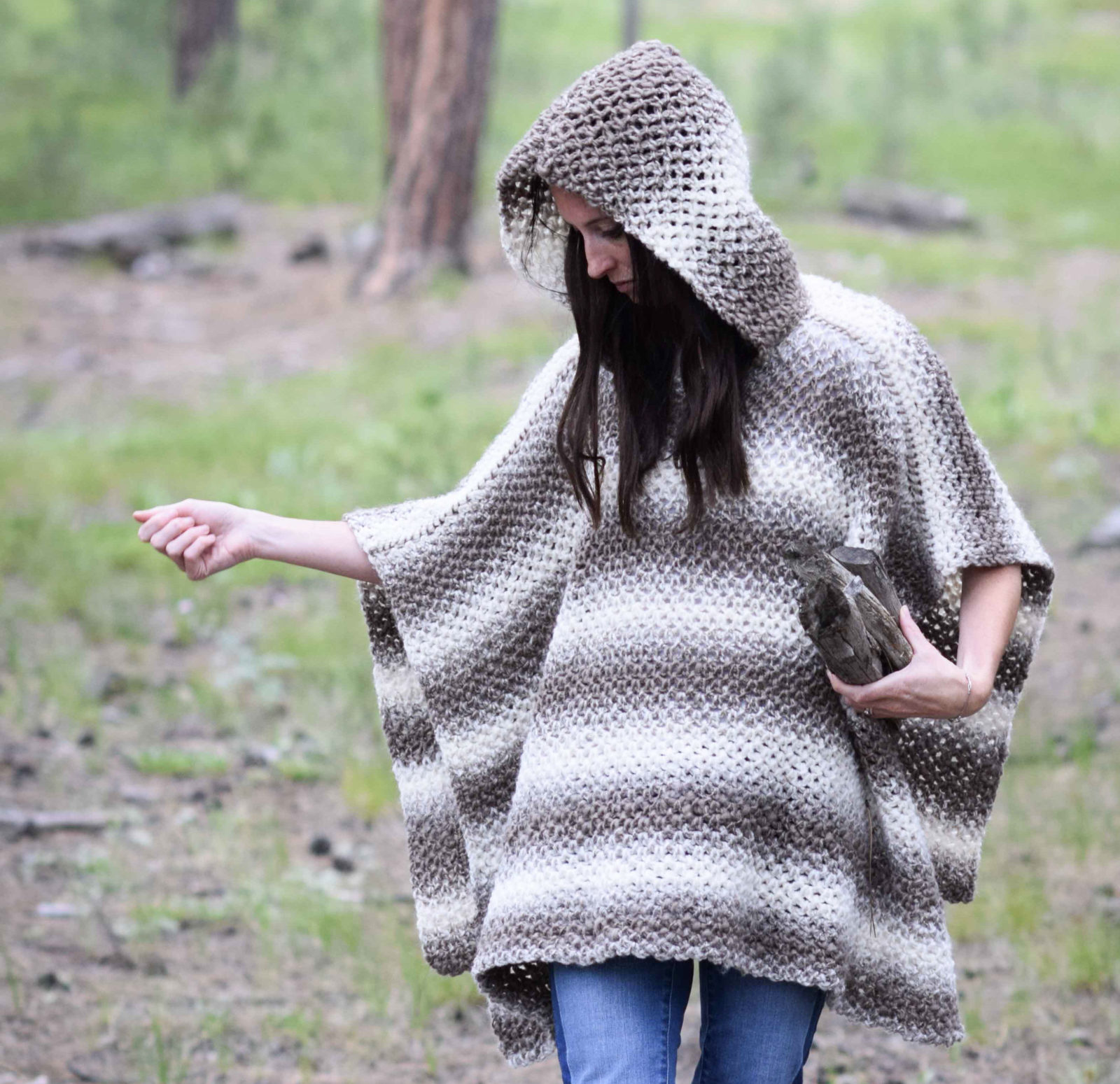This image captures a candid portrait of a woman standing outdoors, likely in a field or a forest with greenery and trees in the blurred background. She is wearing a distinctive woolen poncho, which is white with horizontal grey or dark brown stripes, and it covers her head. The woman has long, dark brown hair and is looking down at the ground. She is holding several pieces of firewood or kindling in her left hand, while her right hand, adorned with a ring and a bracelet, is poised as if she is about to pour something. Her blue jeans add a touch of color to the earthy tones of her attire and surroundings. The composition captures her from just above the knees, focusing mostly on the top half of her body, and the overall feel is one of tranquil simplicity set against a natural, woodsy backdrop.